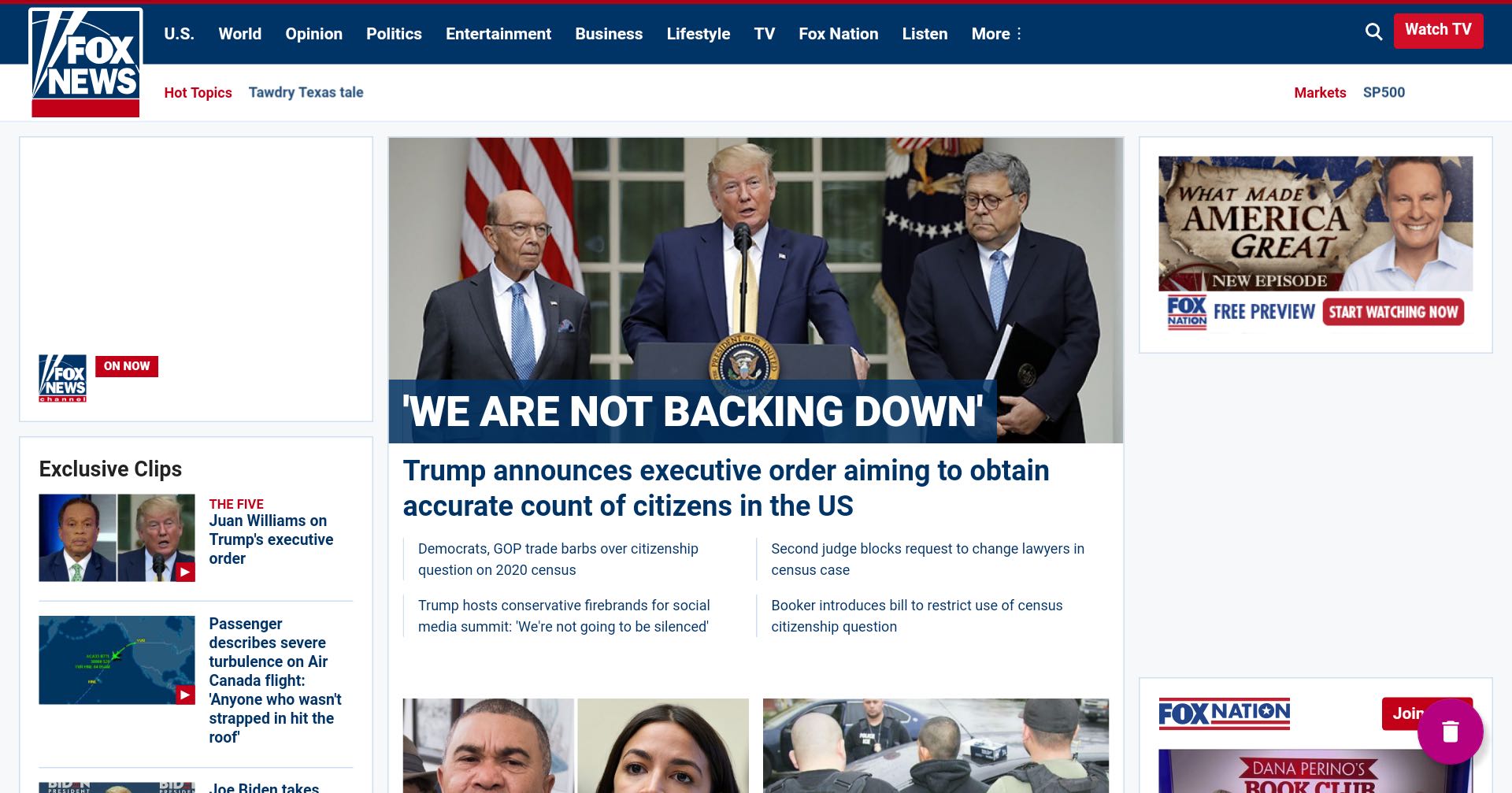Here is a detailed and cleaned-up caption:

---

Screenshot of the Fox News website depicts a dark blue header bar featuring white text links to various sections including US, World, Opinion, Politics, Entertainment, Business, Lifestyle, TV, Fox Nation, Listen, and More. In the top right corner, there are two buttons: one for search and a red "Watch TV" button.

At the top left, the Fox News logo is prominently displayed. Just below the header, bold red text reads "Hot Topics," followed by blue text "Towel Dry Texas Tale." Further right, red text indicates "Markets" while blue text mentions "SP500."

The main content area centers on a large image of Donald Trump with a group of people at a podium. The accompanying headline emphasizes Trump's declaration: "We Are Not Backing Down." The subhead details Trump's executive order to obtain an accurate count of citizens in the US, mentioning opposition from Democrats and GOP as well as highlighting controversies around the 2020 census. Additional news snippets cover Trump's conservative social media summit and legal challenges concerning the census citizenship question, including a judge blocking a request to change lawyers and Booker introducing a bill to resist the use of the citizenship question.

On the left side, a section titled "Exclusive Clips" lists recent segments: Juan Williams on Trump's executive order in 'The Five', a passenger's account of severe turbulence on a Canada flight, and discussions on various incidents.

The right side features a promotional banner with the text "What's Made America Great" promoting a free preview of a new episode with a red "Start Watching Now" button prominently displayed over a red background.